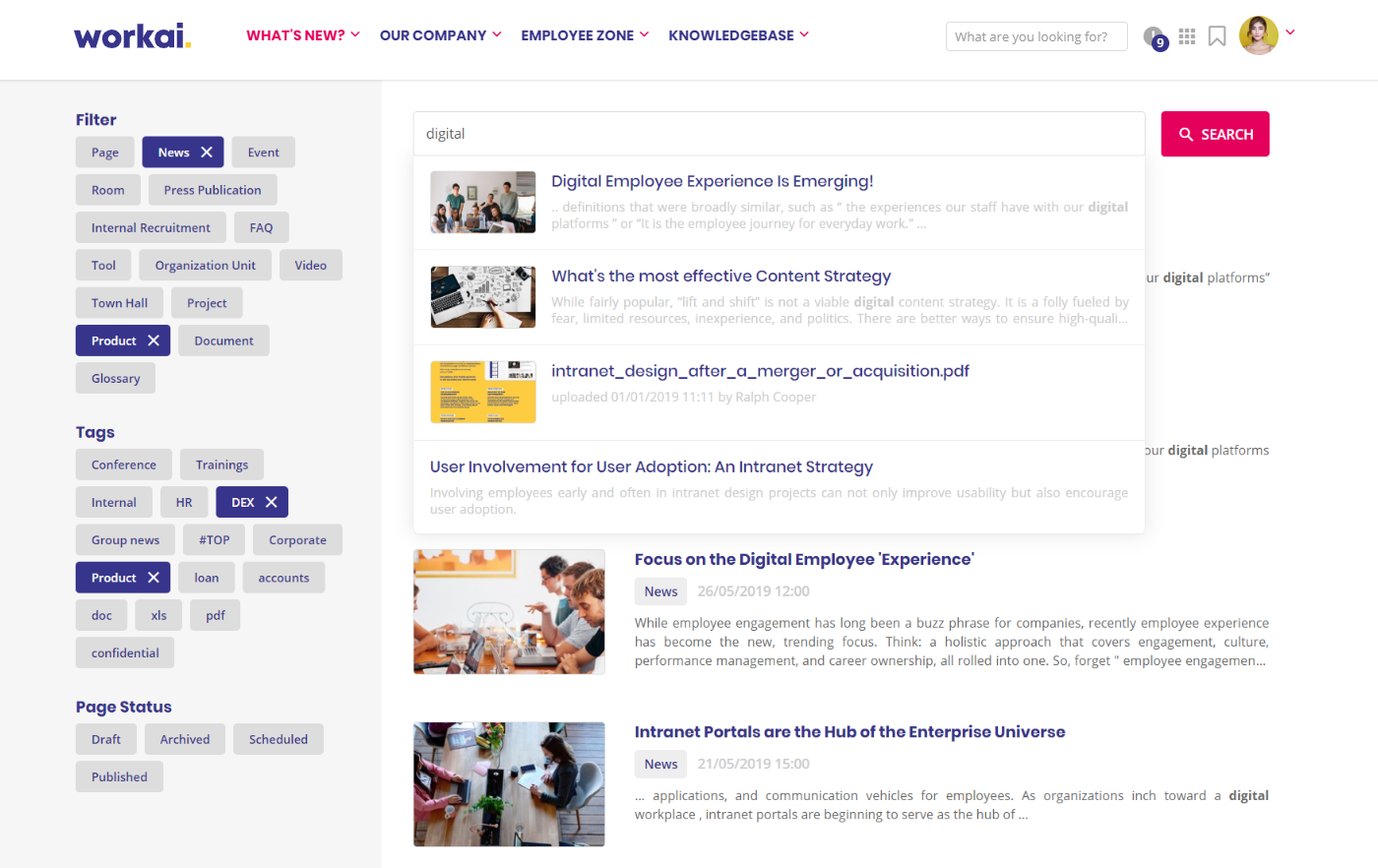A screenshot of a corporate intranet platform titled "Work AI" is displayed. In the top left-hand corner, "Work AI" is prominently shown in dark purple. Adjacent to this, there are several navigation tabs including "What's New?" in pink, "Our Company," "Employee Zone," and "Knowledge Base" all in dark blue.

Running down the left-hand side, there are various filter options encased in gray boxes with dark purple text. The filter choices include: 
- Page (highlighted in dark purple with a white X)
- News
- Event
- Room
- Press Publication
- Internal Recruitment
- FAQ
- Tool
- Organization Unit
- Video
- Town Hall
- Project
- Product (also highlighted in dark purple with a white X)
- Document
- Glossary

Below these filters, another section labeled "Tags" offers further categorization options:
- Conference
- Trainings
- Internal
- HR
- DEX (highlighted in purple)
- Group News
- Hashtag Top
- Corporate
- Product (also highlighted in purple)
- Loan
- Accounts
- Doc
- XLS
- PDF
- Confidential

The final section on the left is labeled "Page Status" and includes these choices: 
- Draft
- Archived
- Scheduled
- Published

The main body of the page features thumbnails of various articles, each accompanied by a title in dark text, a short description in gray text, and a rectangular photograph.